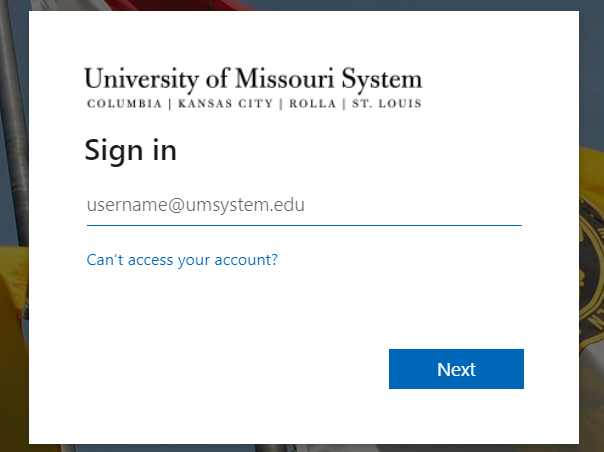Screenshot of the University of Missouri System Sign-In Page: The image is a cropped screenshot focusing primarily on the sign-in section of the University of Missouri System's webpage. The backdrop features a faded image with hints of blue, yellow, and black, possibly depicting a construction site, equipment, a vehicle, or tools, but is indistinct. Front and center on the page is the sign-in box, prominently displaying "University of Missouri System" at the top. Below this, the names of the universities within the system are listed: University of Missouri Columbia, University of Missouri Kansas City, University of Missouri Rola, and University of Missouri St. Louis. There is a field labeled with a placeholder "username@umsystem.edu" for users to enter their email, underlined in blue. Below this field, a hyperlink in blue text reads "Can't access your account?" that users can click if they encounter login issues. At the bottom right corner of the sign-in box is a blue "Next" button.